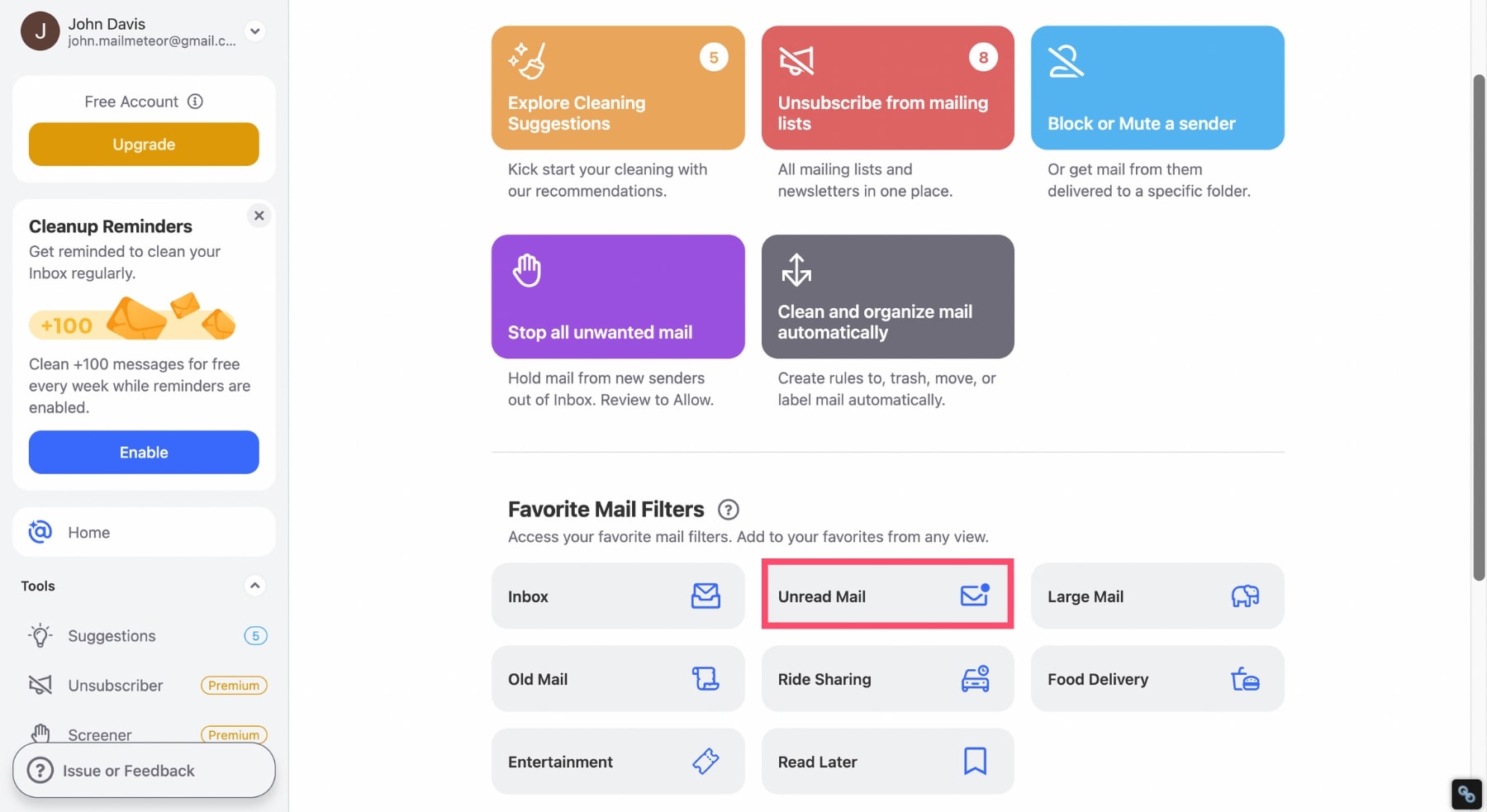Here is a comprehensive and well-structured caption for the described image:

---

The image showcases a screenshot of a Gmail account page belonging to johndavisjohn.malmeteoratgmail.com. At the top of the interface, there is a down arrow next to the account name, along with an indicator stating "Free Account!" accompanied by an orange box labeled "Upgrade." 

Just below, a notification banner suggests users to "Clean up reminders" with a note stating "Get reminded to clean your inbox regularly." This notice includes a gray "X" in the corner to dismiss it.

The main feature highlighted is an image showing "+100" and several mail icons. The accompanying text explains, "Clean 100+ messages for free every week while the reminders are enabled," followed by a blue "Enable" box.

On the left-hand sidebar, several tool options are listed, including:
- Home
- Tools, which expand to reveal:
  - Suggestions (with a number "5" next to it)
  - Unsubscribe
  - Screener
  - Issue or Feedback
  - Unsubscriber
  - Screamer
  (All options except "Suggestions" are marked with a premium icon.)

The right-hand sidebar contains various features, each in different colors:
- Explore Cleaning Suggestions
- Unsubscribe from Mailing List
- Block or Mute a Sender
- Stop All Unwanted Mail
- Clean and Organize Mail Automatically

Towards the bottom of the page, there is a section for favorite mail filters, listing:
- Inbox
- Unread Mail (highlighted in a red box)
- Large Mail
- Old Mail
- Ride Sharing
- Food Delivery
- Entertainment
- Read Later

---

This caption offers a clear, detailed, and organized description of the Gmail account page, making each feature and section easy to understand.